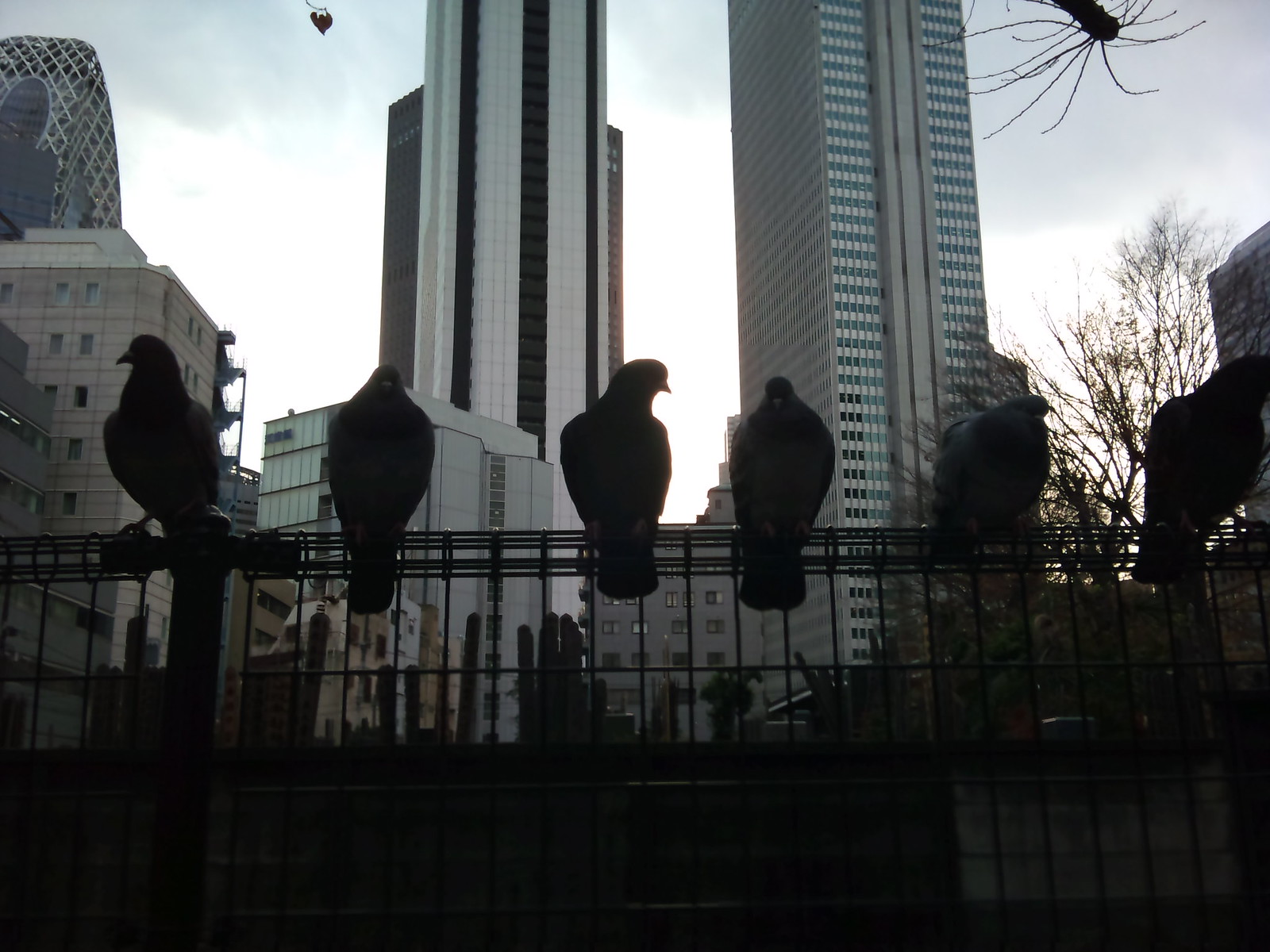This outdoor photograph, likely taken at dawn, captures a somewhat dim, overcast cityscape bathed in the first light of morning. Centered in the foreground is a horizontal wire fence, dark and silhouetted, spanning the width of the image. Perched along the fence are six pigeons, also in silhouette, each facing different directions. Behind them, a pair of tall skyscrapers, along with some shorter buildings, rise up and out of the frame. The skyline is tinged with a dull, grayish hue as clouds obscure the emerging sunlight. In addition to the man-made structures, the upper corners of the image show hints of scraggly tree branches, contributing to the scene's urban texture. The overall mood is serene, with the interplay of dim lighting and silhouetted elements evoking a calm, early morning atmosphere.